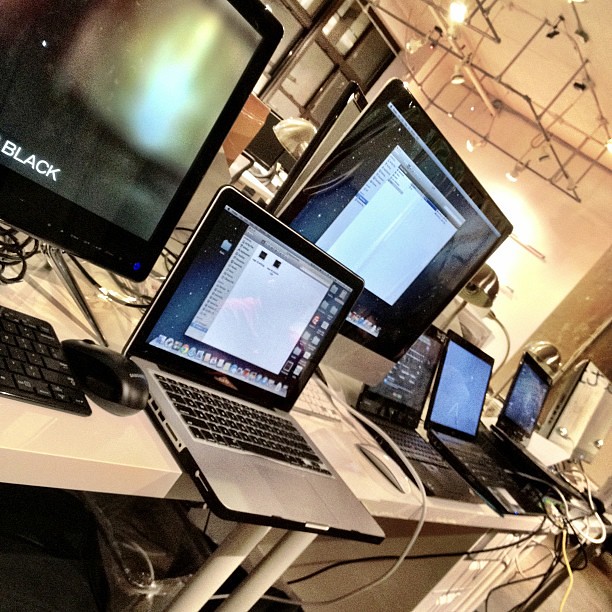The image depicts a large, white room with a steel-like structure supporting circular ceiling lights that are bright and directed toward various workstations. In the foreground, a long, white table with uniquely shaped legs holds an array of computer equipment. There are four laptops on the table: three black and one silver. Two large computer monitors, one with a white trim and another displaying the word “black,” are positioned centrally on the table. The table is cluttered with various peripherals including multiple keyboards, a white and a black mouse, and an abundance of wires in black, yellow, and white colors. Additionally, a clear plastic bag is noticeable under the table on the left-hand side. The setting appears to be some type of office or gaming room, featuring visible steel beams and pipes running along the ceiling with attached lights that have white housing and emit a yellow glow. The laptops and monitors display different computer programs, contributing to a busy and tech-centric atmosphere.